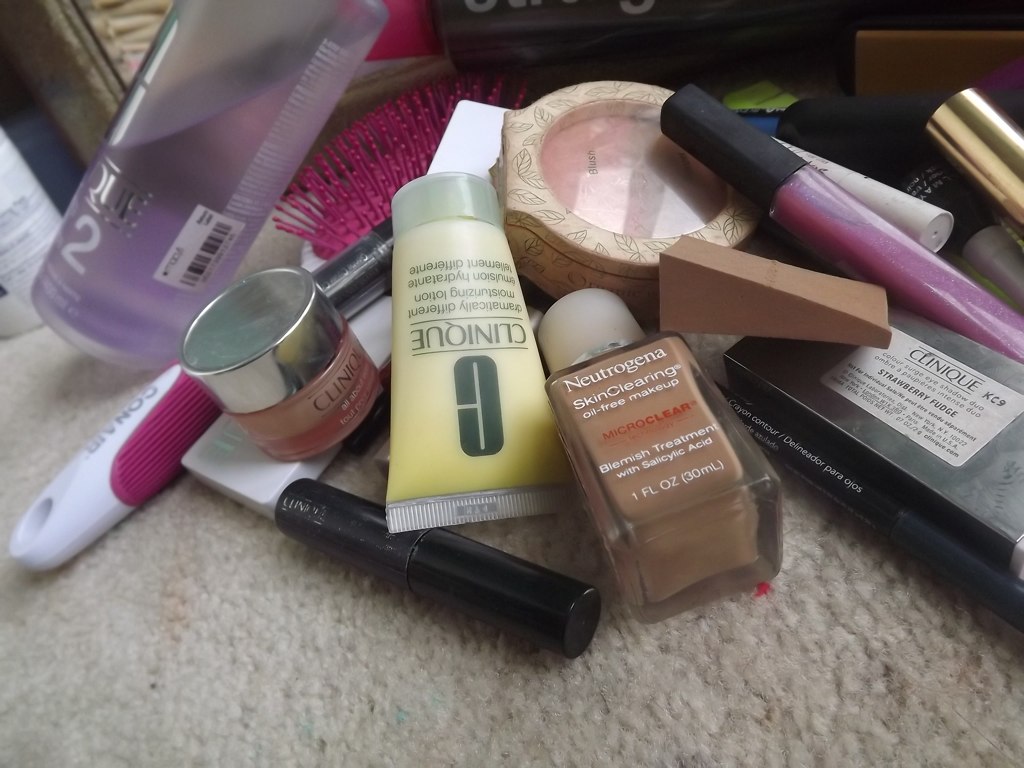This close-up image showcases an assortment of over a dozen beauty products strewn across a slightly dirty beige carpet, which features various colorful stains suggesting past spills. 

Starting from the top left corner, a sideways bottle filled with purple liquid prominently displays the number "2," though its other text is illegible. Next to it lies a pink and white brush branded "Conair." Below this brush, there's a small brown bottle with a silver cap, labeled "Clinique." Underneath the Clinique bottle, an indistinguishable white object can be seen. 

Further along, there is a black tube with no visible writing and an upside-down yellow tube also bearing the "Clinique" label. Nearby, a bottle of Neutrogena SkinClearing Oil-Free Makeup with MicroClear Blemish Treatment and Salicylic Acid (one fluid ounce or 30 milliliters) is seen. The collection also includes a black eyeliner pencil and a brown Beauty Blender. 

Amidst the others, there is a cylindrical container likely holding blush or bronzer and a tube of pink lipstick with a black cap. An additional unidentified white tube is present. Completing the assortment, a black box on the right side of the image is labeled "Clinique Strawberry Fudge."